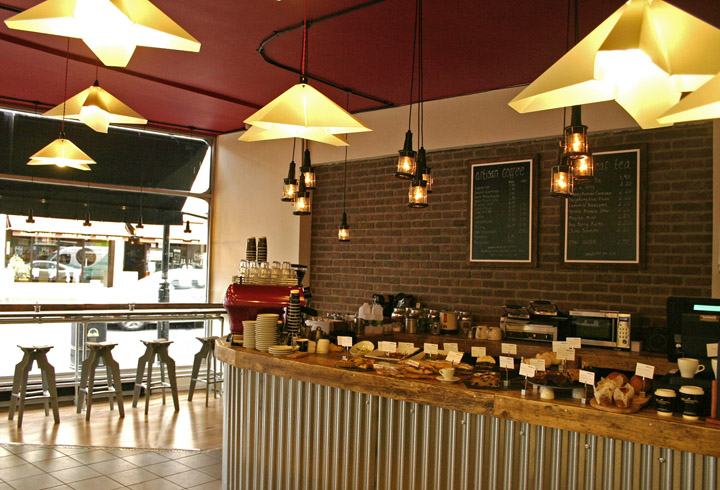The image depicts the interior of a vibrant and up-to-date restaurant bistro with elements that suggest it could also be a bakery or coffee shop. The space features low ceilings painted a bright red, adorned with track lighting pipes. Various types of hanging lights are suspended at different lengths, including clusters of lantern-like fixtures and a mix of fancy Edison bulbs. Some lights have yellow shades, while others are star-shaped with bright white lighting.

A striking brick wall dominates the right side, showcasing two green chalkboard menus framed in brown wood with white borders, detailing menu items and prices. Below the menus, a countertop displays an array of food items, including pastries, a microwave, plates, cups, and a coffee maker.

The bar area is a focal point, with its front finished in variegated tin and a thick wooden base that curves gracefully. Additional seating is available at another bar along a window that faces the street. Through the clear glass window, a dark green awning is visible, and four stools are lined up, offering a cozy spot for patrons to enjoy their drinks and treats. The overall atmosphere is a blend of modern sophistication and welcoming warmth.